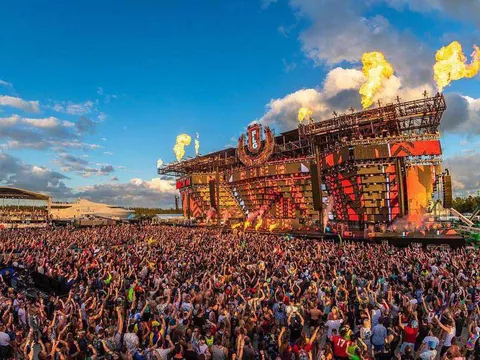The image captures an extravagant outdoor music event, teeming with thousands, if not hundreds of thousands, of attendees. Set against a bright blue sky dotted with clouds, the scene is dominated by a massive, elaborate stage constructed of wood and illuminated in vibrant hues of reds, browns, and yellows. Crowning the stage is a large sign bearing the vertical letters "F.L.G.," nestled within a horseshoe-shaped structure. Fiery pyrotechnics erupt from the stage, with four distinct balls of flames adding to the dramatic atmosphere. Although the crowd, waving their arms and seemingly applauding, obscures any performer, the festive energy is palpable. To the left, a tent-like pavilion—possibly a VIP or medical tent—adds to the venue's amenities. The overall setup suggests a grand, remote festival reminiscent of iconic events like Coachella or Burning Man.